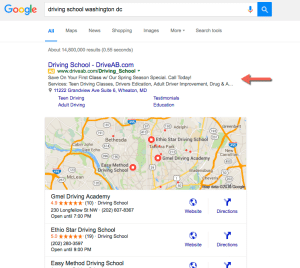The image is a vertical, rectangular screenshot of a Google search results page with a light gray background. At the top of the image is the Google search bar, which is rectilinear and white with the word "Google" on the left, displayed in multi-colored letters. Inside the search bar, in black lowercase font, are the typed words "driving school Washington DC". To the right of the text in the search bar is a small microphone icon followed by a turquoise square containing a white microphone symbol.

Beneath the search bar are small navigational menu items. The first menu item, highlighted in turquoise with an underline, reads "All". To the right of it are additional options labeled "Maps" and "News", though other menu items are too small to be discerned clearly.

Below this menu is a line displaying the number of search results. Further down, the actual search results begin. The first result is presented in a blue-purple, bold font, reading "driving school - driveAB.com." A red, bold arrow on the right side points toward this entry. Under this entry, a small horizontal map appears, featuring three points marked by white dots encircled in red.

Following the map are three additional listings of driving academies, with the first one named "GMEI Driving Academy", and the other two entries featuring names of other driving schools. The image meticulously details the features of a search engine result page for driving schools in Washington DC.